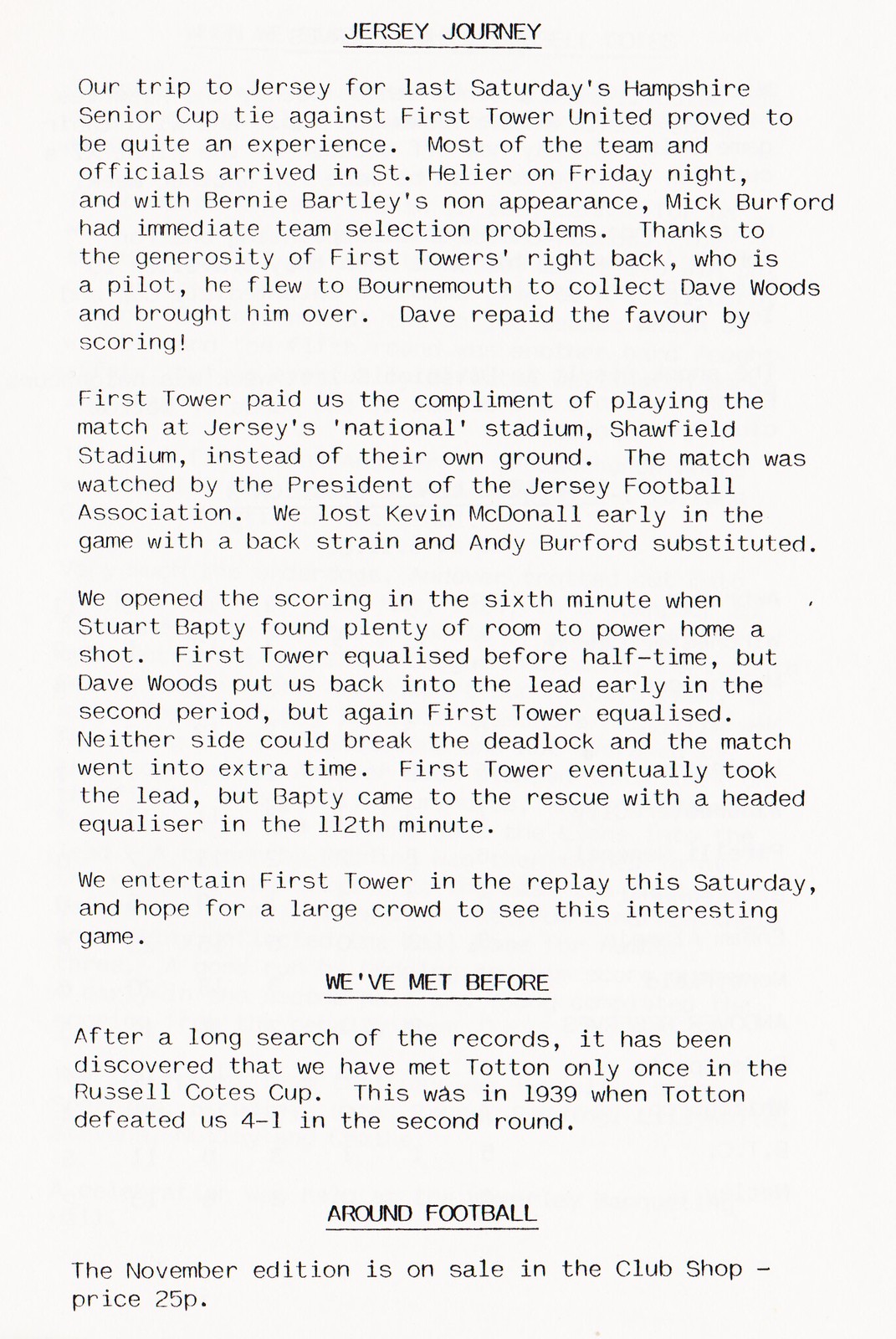This image features a scanned page, possibly from a book or newspaper, filled with black text on a white background. The text spans the entire image and is divided into three sections. The first section, titled "Jersey Journey," comprises four paragraphs. It narrates the team’s trip to Jersey for last Saturday's Hampshire Senior Cup tie against First Tower United, highlighting the experience as eventful. Most of the team and officials arrived in St. Helier on Friday night. Bernie Bartley's absence posed immediate team selection problems for Mick Burford. However, thanks to the generosity of First Tower's right back, who is a pilot, he flew to Bournemouth to collect Dave Woods, who repaid the favor by scoring. The match was held at Jersey's National Stadium, Sheffield Stadium, instead of First Tower's home ground, and was attended by the president of the Jersey Football Association.

The second section is titled "We've Met Before" and reveals that after a comprehensive search of historical records, it was found that the team had previously played against Totten only once, in the 1939 Russell Coates Cup second round, where Totten won 4-1.

The final section, labeled "Around Football," consists of a single sentence: “The November edition is on sale in the club shop. Price 25p.”